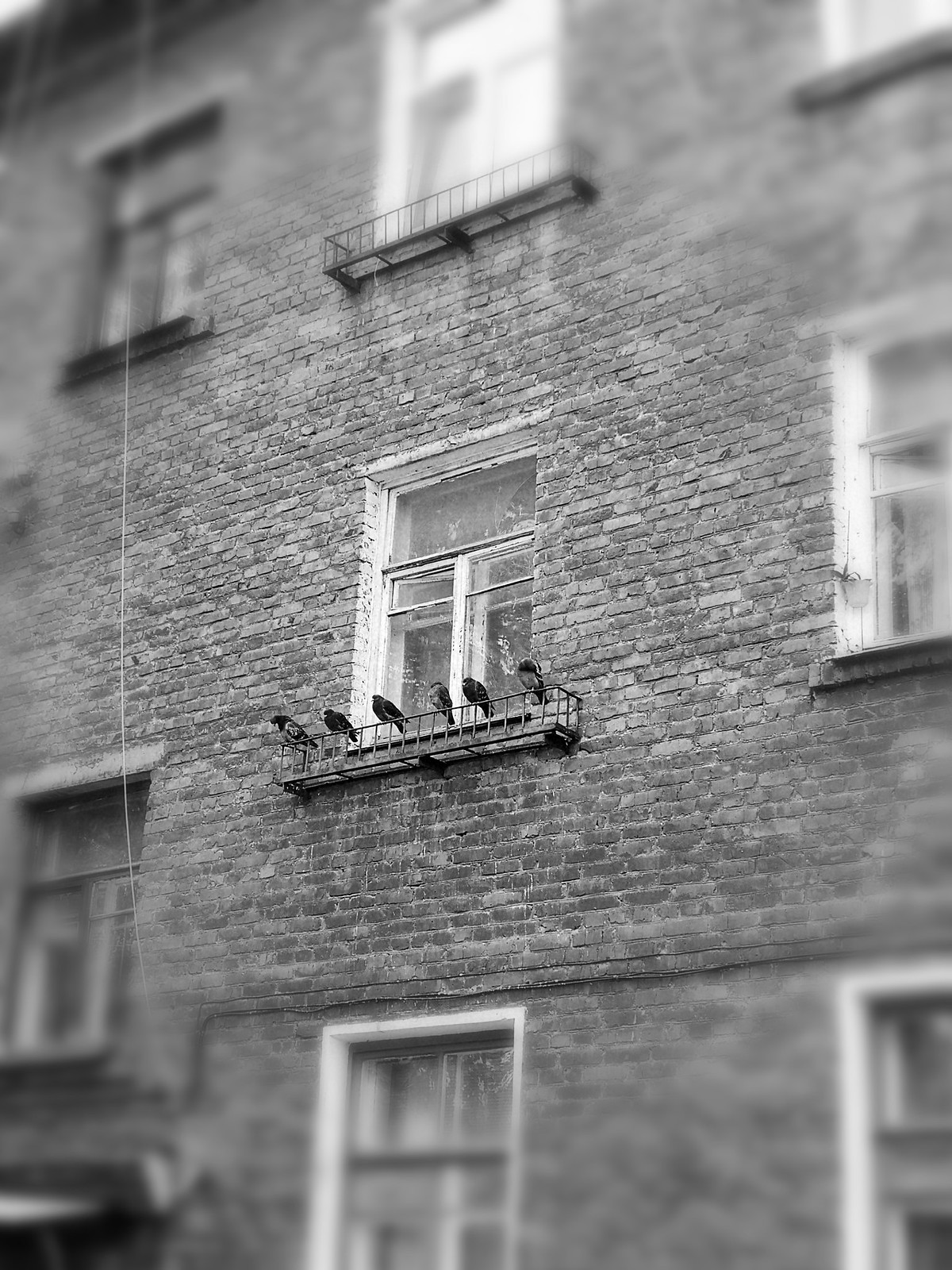This black-and-white photograph captures the side of an apartment building, taken using a tilt-shift technique that sharply focuses the center of the image while blurring the edges. The building’s brick exterior is prominently featured, along with several windows. The central focus is on a three-paned window with a rectangular top pane and two vertical rectangles below it, where six pigeons are perched on the metal windowsill, all facing towards the left. Above this window, another one with a similar metal outside rack remains empty. The image, taken in daylight, presents a crisp and detailed view in the center, making the pigeons the focal point amidst the slightly blurred peripheral windows and brickwork.